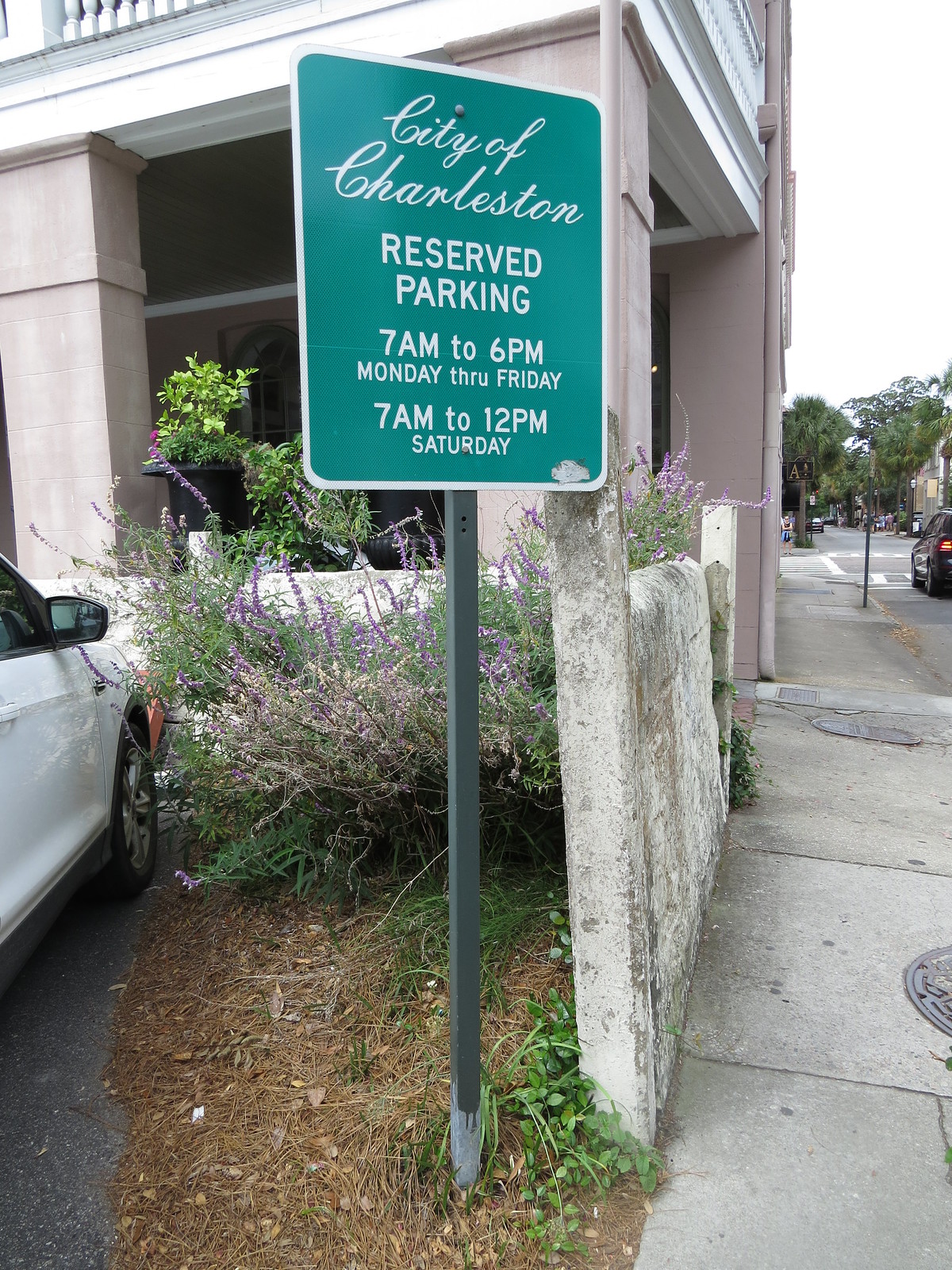This photo captures a green sign with a white outline, prominently displaying the text "City of Charleston" in white. Below it, the sign outlines parking regulations: "Reserved parking 7 a.m. to 6 p.m. Monday through Friday, 7 a.m. to 12 p.m. Saturday." The sign is mounted on a gray pole that has a slightly silver base where it anchors into the ground, surrounded by old leaves and brush. Behind the pole, there's a mix of wild green and purple bushes and flowers that add a natural, untamed backdrop. To the left, a white car is partially visible. A building stands farther behind the sign, with a short wall extending in an L shape alongside the parking area. The image also includes a sidewalk with sewers running parallel to a street on the right. The distant trees and the cloudy sky contribute to the overcast ambiance of the scene.